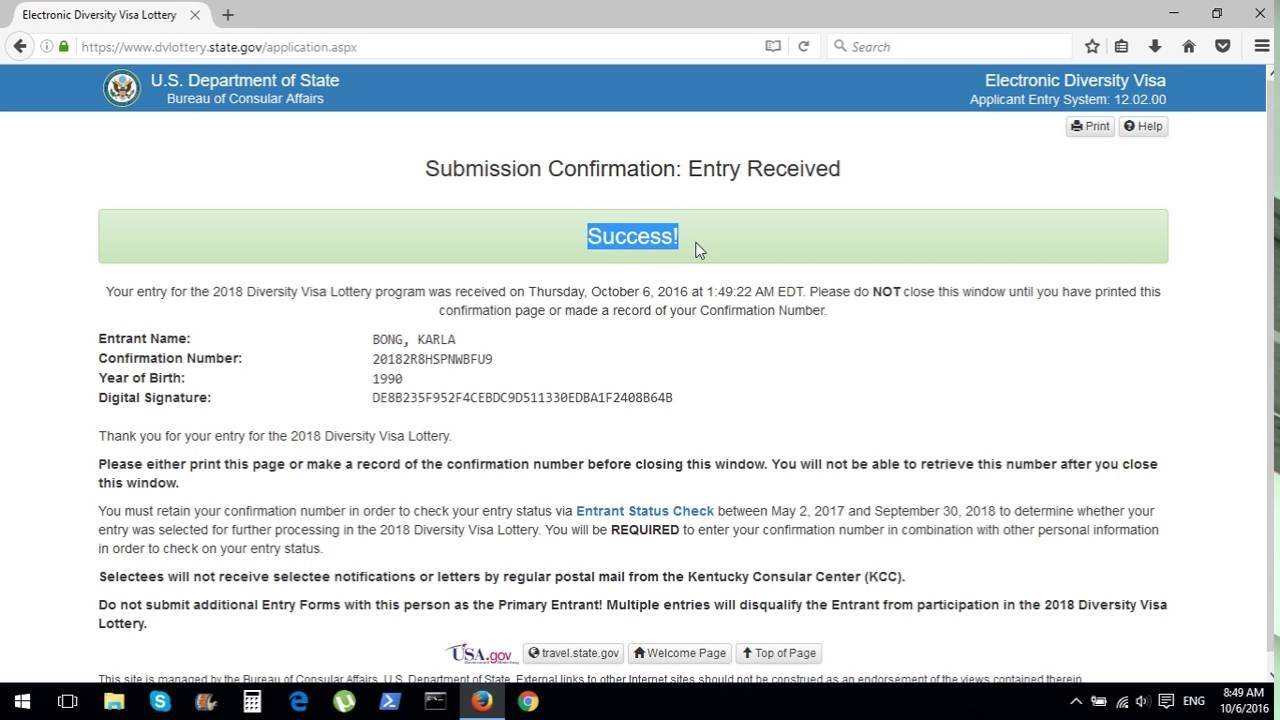The image displays a computer screen capturing what appears to be a webpage from the U.S. Department of State related to the Electronic Diversity Visa program. 

At the very top of the screen, there's a light gray background section where the browser controls are visible, including minimize, maximize, and close buttons. Beneath this is the browser URL bar, which includes the website address on the left and a separate search bar to its right, followed by six icons: a star, a square, a downward arrow, a home icon, a shield-like shape with a downward arrow, and a three-line tab menu.

The main section of the webpage has a blue background header that reads "U.S. Department of State," with "Electronic Diversity Visa" to its right. Below this, the text "Submission Confirmation Entry Received" is displayed. Centrally located on the screen is the word "Success" highlighted in blue with a green rectangle around it, and the computer mouse pointer is positioned directly to the right of it.

Further down, four categories are listed: "Entrant Name," "Confirmation Number," "Year of Birth," and "Digital Signature," with their respective information provided to the right of each category. At the bottom segment of the screen, some black text sentences present additional information.

Finally, the bottom-right corner of the screen features several computer system icons, including the time, a Wi-Fi symbol, and a battery indicator.